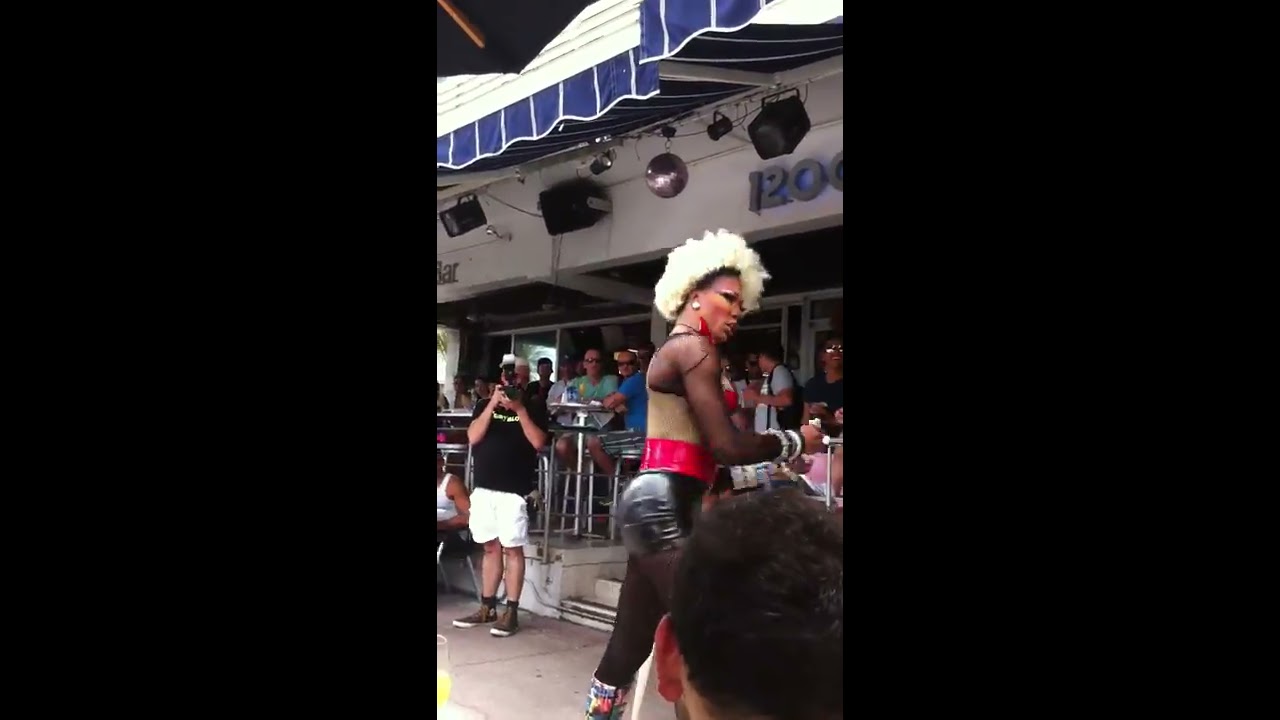The image depicts a lively outdoor scene, possibly at an open-air bar or restaurant marked by the address 1200 on a white building adorned with a blue canopy. The central figure, whose gender is ambiguous, captures attention with striking attire and appearance: short black leather shorts, a tan or white tight-fitting tank top, a red wrap or belt around the waist, and a voluminous white or blonde wig. This person is adorned with earrings and heavy makeup, contributing to a dramatic look suggestive of drag. They are positioned side-on, gazing to the right, while in the background, a mix of seated patrons at high silver tables and an individual in a black t-shirt and white shorts actively taking a photo with a camera add to the animated atmosphere. The scene is framed with thick letterbox bars on both sides, lending a cinematic quality to the image.